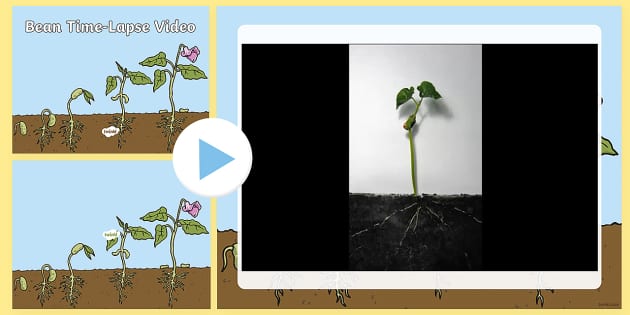The image is a detailed and multi-layered graphic depicting the growth stages of a bean plant, presented in a time-lapse video format. It features a thin yellow border around the entire image, enhancing its visual appeal. The content is divided into three main sections. On the left side, there are two smaller horizontal rectangles, one stacked on top of the other, each with a yellow border and a blue background. Both rectangles are labeled "Bean Time-Lapse Video" in a playful bubble lettering style and contain cartoon illustrations showing the stages of bean growth, with each stage depicted above a patch of brown dirt. The top rectangle shows five distinct stages of growth, including a small green stalk emerging from the dirt, progressing to various stages until a mature plant appears, accompanied by a white tag beneath the fourth stage. The bottom rectangle presents a similar sequence, with a white tag positioned at the top of the fourth stage and a play button indicative of video content.

On the right side, occupying the majority of the image, is a depiction of a real bean plant on a white iPad or tablet with a black screen. This section shows the final stages of the bean's development, complete with visible root systems extending into the black dirt. Above this image is a white circle with a blue arrow pointing to the right, resembling a play button, indicating that this is video content. The entire presentation effectively contrasts the animated growth stages with the real-life development of the bean plant, providing a comprehensive and visually engaging representation of the bean's growth process.